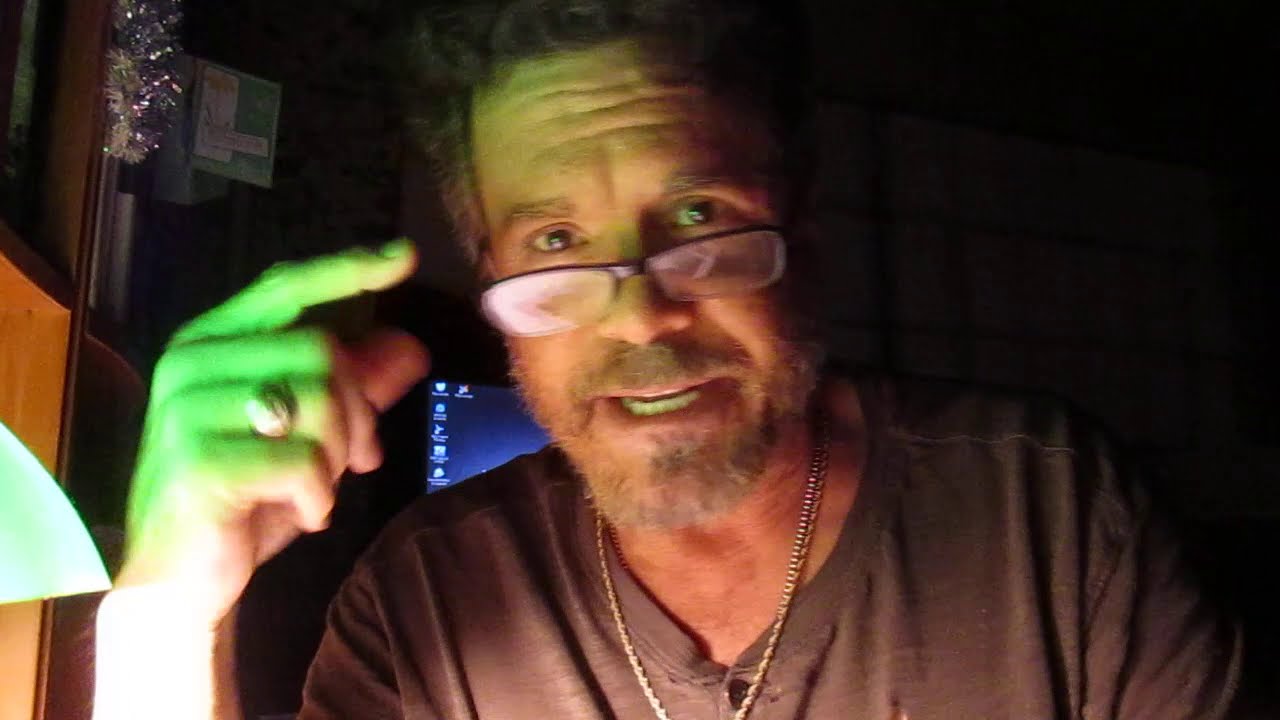The image captures a white male, likely in his late 40s or early 50s, sitting in an office or home office setting. The man is looking directly into the camera, suggesting it's a webcam capture or a screenshot from a Zoom meeting. He has thick, brown wavy hair with gray at the sides and a full gray beard. He’s wearing black-framed reading glasses at the tip of his nose, and two silver chain necklaces around his neck. He is dressed in a gray, V-neck shirt with buttons at the top. His right hand is raised, pointing upwards to the left of the image, showcasing a silver ring on his finger, illuminated by green light from a desk lamp with a green lampshade in front of him. Behind him, the room appears moderately lit and features a computer monitor with icons, a wooden bookshelf with books, and some curtains possibly covering a window. There are also some Christmas decorations on the right side of the wall.